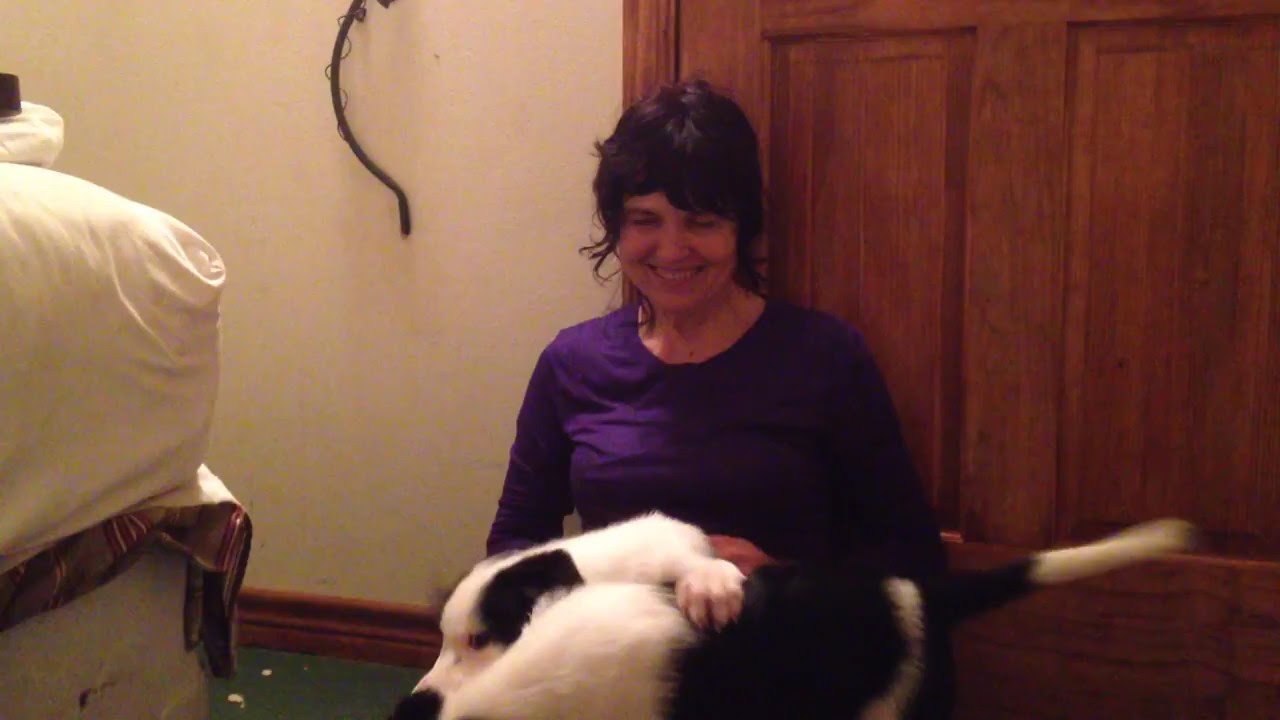In this warmly lit living room photograph, a smiling woman in her 30s with slightly disheveled, short black hair, sits comfortably on the green-carpeted floor in front of a dark wooden door. She is wearing a high-neck purple shirt and holding a black and white dog on her lap. Another black and white dog with distinctive dark ears and a dark nose is situated nearby, its paw resting on the back of the dog on her lap. To the left of the door, a white wall features a metal rod or handle. A large white pillow rests on an easy chair to her right, adding a cozy touch to the setting. The overall ambiance of the image conveys a sense of contentment and homey warmth.